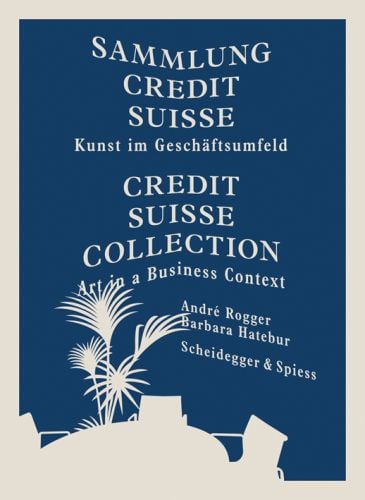The book cover, featuring a predominantly dark blue background with a gray border, introduces itself with a centered title in German, "Sammlung Credit Suisse: Kunst in Geschäftsumfeld," directly translated underneath to "Credit Suisse Collection: Art in a Business Context." This title is succinctly laid across the middle of the cover, ensuring clear visibility. Below the title, the authors are listed as André Roger, Barbara Heber, Scheidegger, and Spies. Complementing the textual elements, a simple yet illustrative drawing occupies the left-hand corner, depicting a table surrounded by three chairs and a plant with multiple palm fronds. The table is centrally placed with one chair on each of the top, left, and right sides, giving a balanced and inviting impression. The plant's fronds stretch towards the text, slightly merging with the letters, adding a touch of organic interaction to the otherwise structured design.